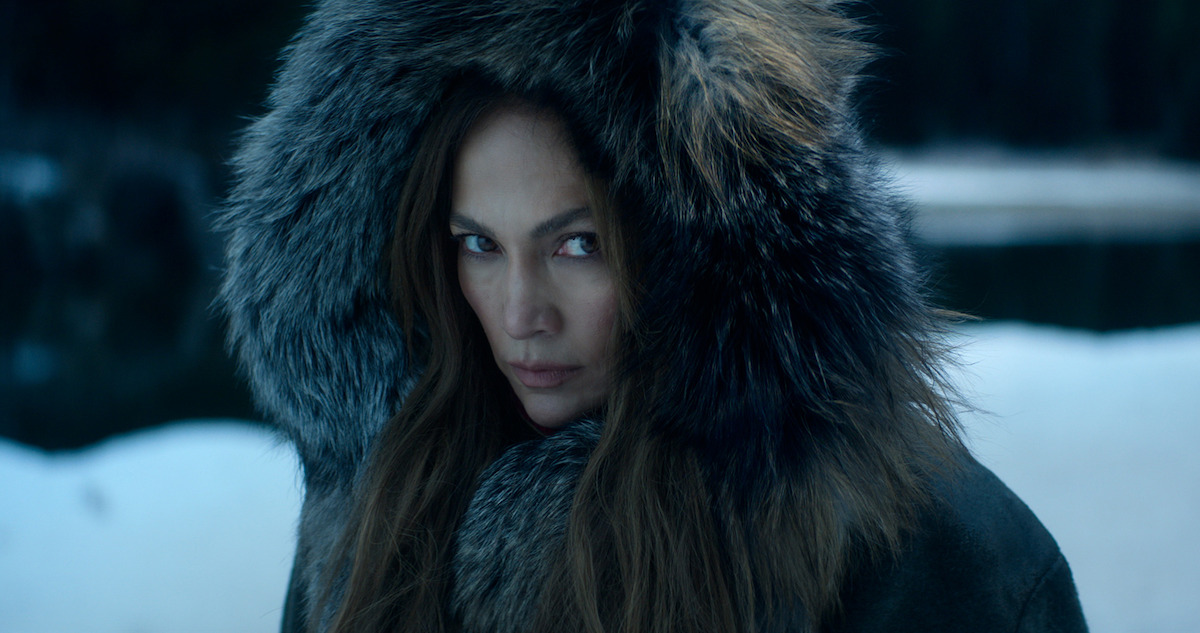In this color photograph with a landscape orientation, actress Jennifer Lopez stands at the center with a worried expression, gazing slightly upward at the viewer. She wears a large black parka-like coat with a hood that is lined with long, shaggy fur in shades of brown, white, and grey, extending around her face and down the front of her coat. Her scarf, matching the hood's fur, adds to the cold, Arctic-like atmosphere. Her face appears flushed from the cold, devoid of makeup, and her eyes dart off to the side, revealing a sense of tension. The snow-covered background is out of focus, enhancing the emphasis on her character, possibly from a scene in "The Mother." The overall lighting is dark, with deep shadows on either side, contributing to the dramatic and chilly ambiance of the image.